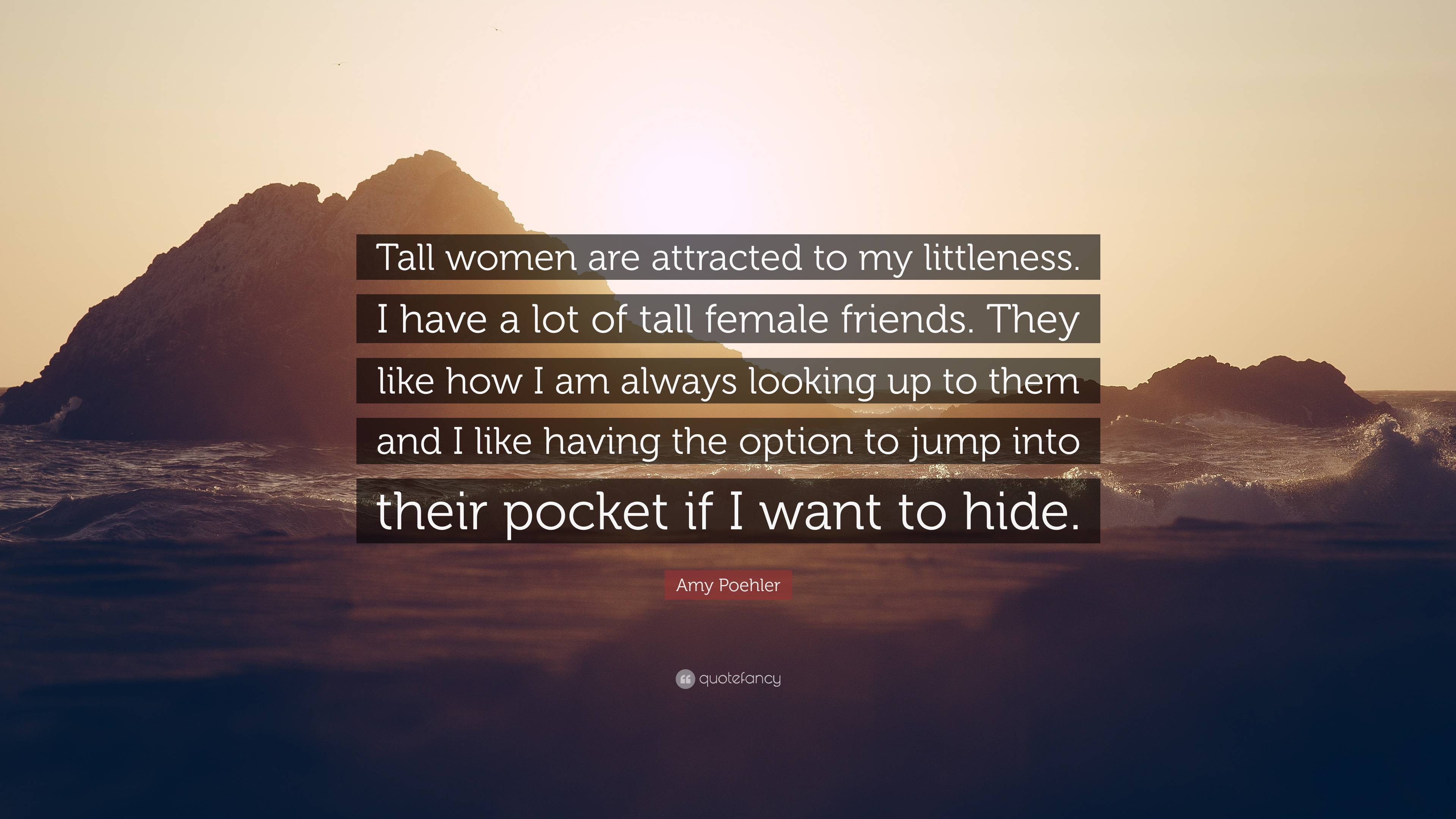The image depicts a rocky beach scene at sunset, with a prominent mountain on the left appearing to jut out from the ocean. The foreground features turbulent waters splashing against the rocky shore. The sky is a hazy light orange hue as the sun sets near the top center. In the middle of the image, white text is superimposed on semi-transparent dark gray rectangles. The text reads: "Tall women are attracted to my littleness. I have a lot of tall female friends. They like how I am always looking up to them, and I like having the option to jump into their pocket if I want to hide." Below this quote is a red rectangle bearing the name "Amy Poehler," and further down, smaller white text reads "quote fancy." The overall color palette of the landscape is dominated by dark silhouettes with only faint hints of brown and orange as the light from the sunset fades.